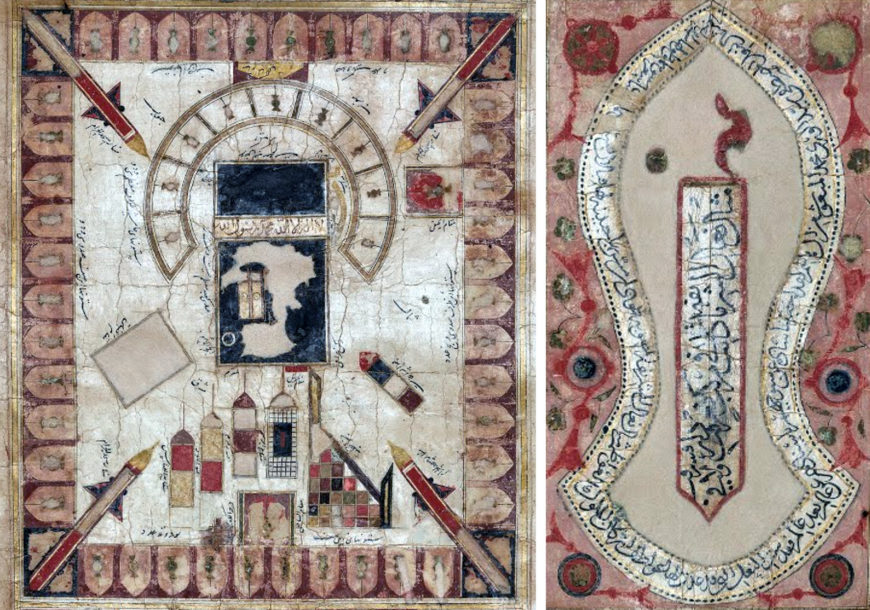This image features two adjacent panels that appear to be ancient or antique, possibly depicting historical illustrations or designed as fabric items like carpets. The left panel, which is wider, showcases a square central area surrounded by various intricate patterns. It features a white center with a border of small squares, blue sections with what appear to be long, pointed shapes resembling rockets or aircraft, and a curved section adorned with tiny points. The perimeter of the left panel is adorned with a repeating pattern of red and pink elements.

The right panel, narrower and more rectangular, has a pink background featuring diamond and square shapes. At its center, there is a beige oval shape interspersed with a long, pointed form and accented by a red tassel-like detail. This panel also includes black symbols or foreign characters, adding to its complexity. Both pieces boast an aged patina, reinforcing their ancient and historically significant appearance.